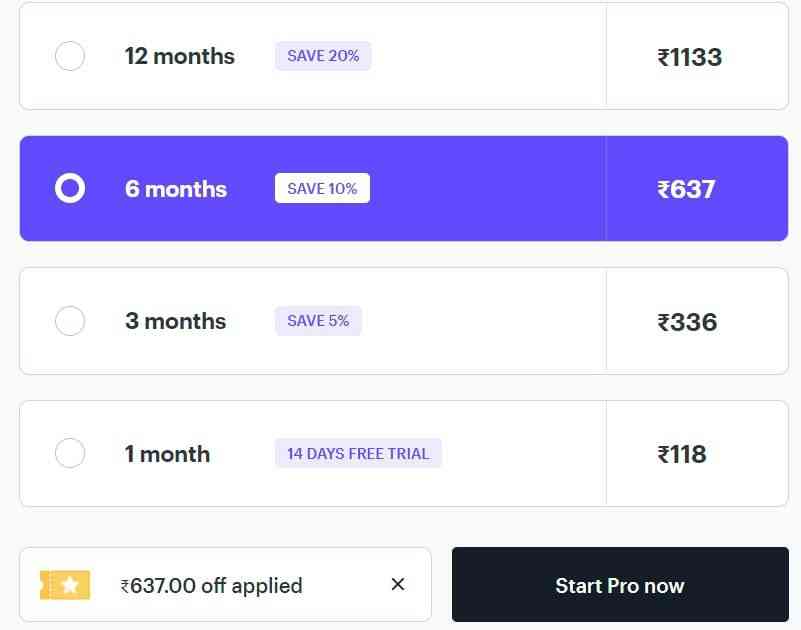This screenshot appears to depict a subscription plan selection interface, possibly from either a mobile device or a computer, but the source device remains unclear. The image, which is roughly square, features a primarily white background divided into four horizontal bars, each representing a different subscription option. 

At the top, the first bar lists a "12 months" plan that offers "20% savings" and is priced at 1,133 in an unidentified currency. The second bar, highlighted in blue indicating it is currently selected, describes a "6 months" plan with "10% savings" for 637 in the same currency. Below this, the third bar presents a "3 months" option that saves "5%" and is priced at 336. The final bar outlines a "1 month" plan, offering a "14-day free trial" for a price of 118. 

Situated below these options are two buttons: The left button is white with text indicating that a "$637 off coupon" has been applied, while the right button is black with the text "Start Pro Now" in white.

Overall, the image provides a clear view of varied subscription lengths and their respective discounts and prices, along with actionable buttons for proceeding with the selection.